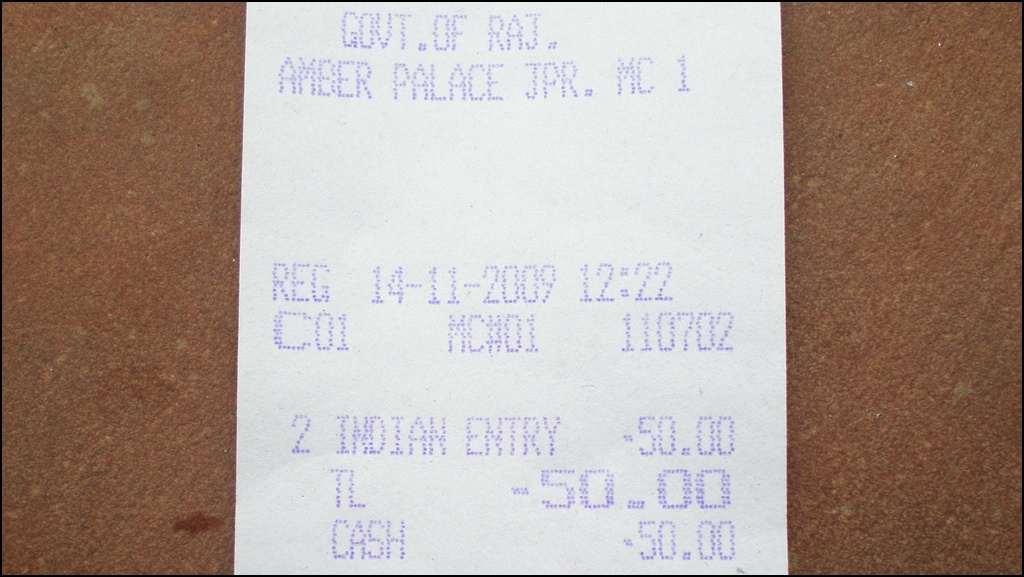**Descriptive Caption:**

A detailed image of a register receipt from an event ticket purchase. The top of the receipt lists "Govt. of Raj." followed by "Amber Palace" and "JPRMC1." The date and time stamp shows that the transaction occurred on November 14, 2009, at 12:22 PM. Below, the receipt indicates an entry fee of $50 for an event labeled "Indian," suggesting an Indian cultural event or visit to a historical site. The total amount paid is $50 in cash. The receipt is photographed against a brown background, which could either be a clipboard or a tabletop surface.